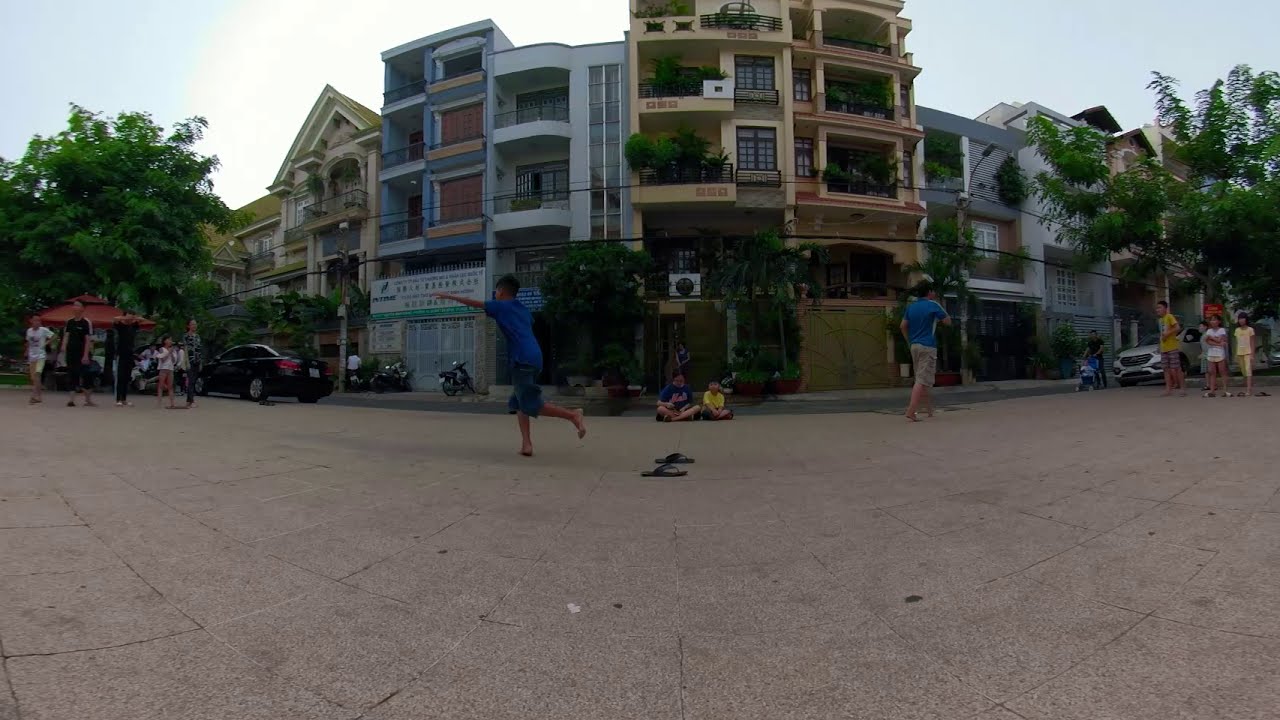This daytime outdoor photograph captures a lively street scene with a slight fisheye effect. In the center, a barefoot boy in a blue t-shirt and denim shorts sprints to the left, leaving his black sandals behind on the brownish-gray cinder block pavement. Another boy, also barefoot, walks in the opposite direction to the right. Near the road, two children sit on the edge of the courtyard, while other kids watch from both sides. On the far right, a group of children observes the scene, and on the far left, a few adults stand near a black sedan parked on the walking area. Behind the open space, marked by the pavement, is a narrow street lined with residential buildings featuring balconies adorned with plants. The sky above is blue with a few wisps of white clouds, indicating a clear, sunny day, creating a crisp yet slightly hazy atmosphere.